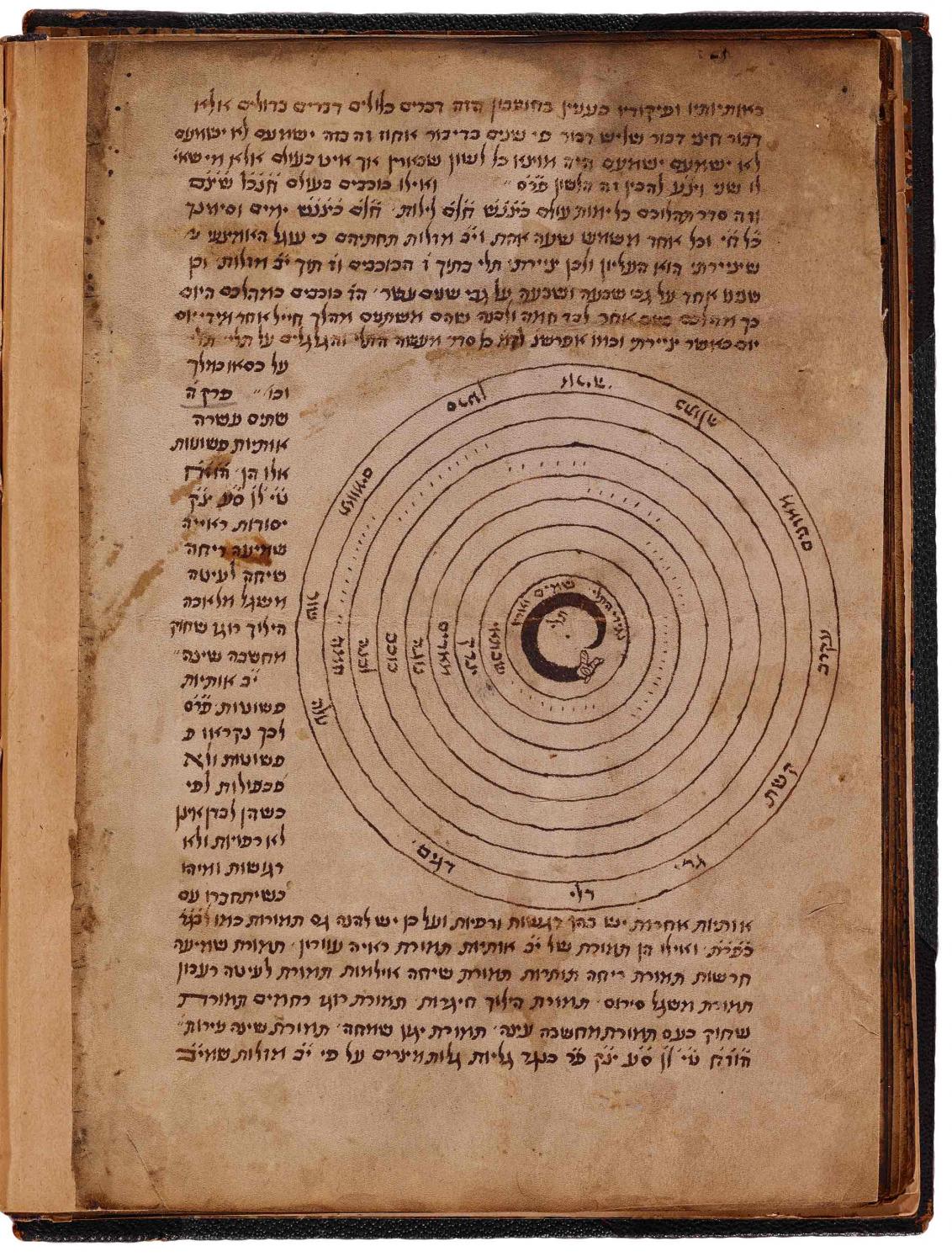The image displays a singular page from what appears to be an old, worn book, likely aged over time, with a brown, water-stained surface. The writing on the page is in a language that is not English and is predominantly spread across the entirety of the page. Central to this page is a peculiar diagram featuring a series of concentric circles, totaling ten in number, each circle contained within the next. The circles become progressively smaller towards the center, creating ring-like formations. Each of these rings contains a word, possibly in the unknown language, arranged in a manner that culminates in a noteworthy dark round ring at the innermost part, which seems to depict a tail-chasing design. Besides the words circling the diagram, there are also dots present within the rings. The diagram disrupts the writing on the left side of the page but remains an integral part of the overall composition. The text and the diagram are inked in black, contrasting against the aged and damaged paper, further emphasizing the historic and possibly significant nature of the book.